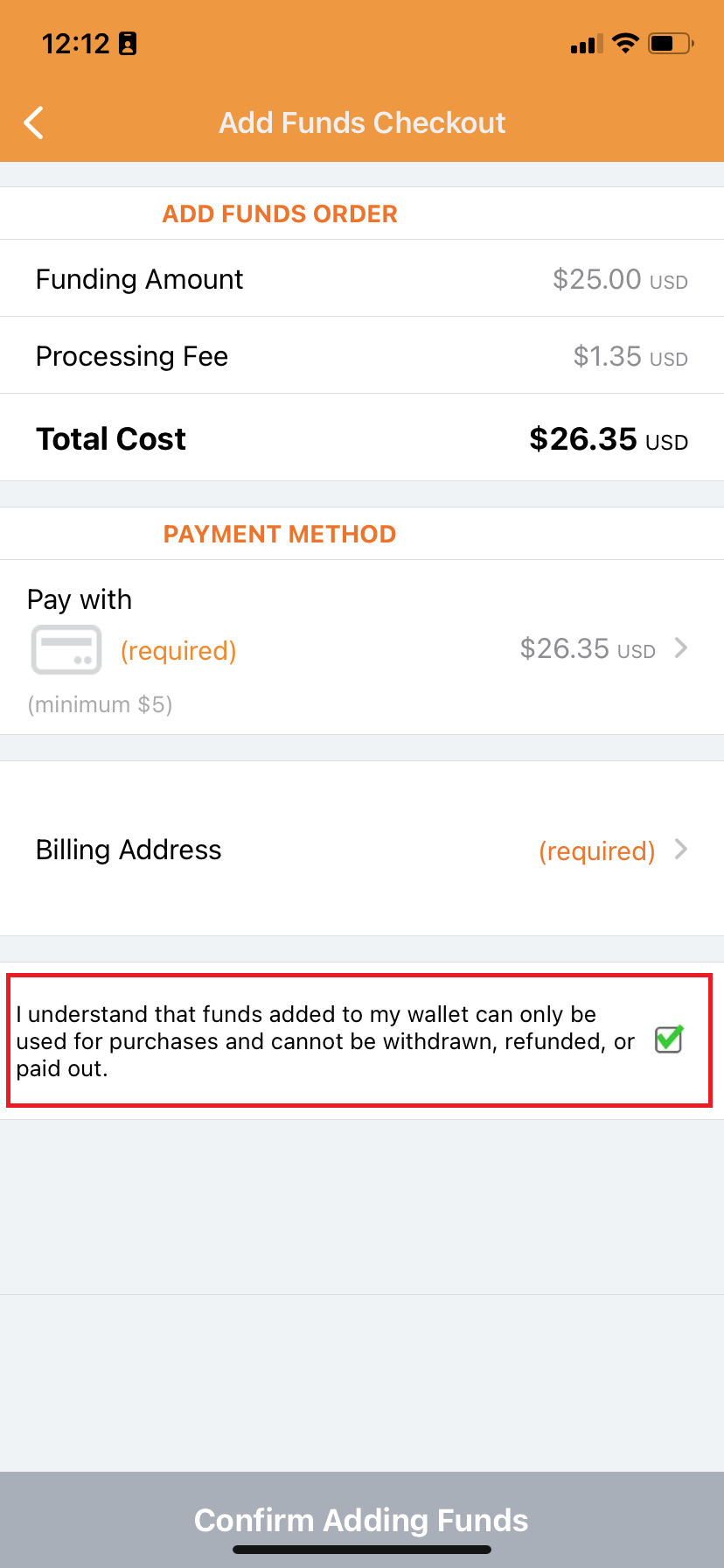Screenshot of a mobile app interface displaying the "Add Funds Checkout" screen. At the top, a prominent thick orange bar reads "Add Funds Checkout." Directly below, the screen details the transaction under "Add Funds Order," showing a payment amount of $25 USD, a processing fee of $1.35, and a total cost of $26.35. Further down in another orange section labeled "Pay With," there's an icon of a credit card indicating that payment is required, with a note specifying a minimum payment of $5. The payment button below this bears the label "Pay $26.35 USD." Subsequently, the app requests a billing address, marked as required. Towards the bottom, there's an outlined red box indicating the necessity to agree to terms with a checked mark confirming agreement. This text reads, "I understand that funds added to my wallet can only be used for purchases and cannot be withdrawn, refunded, or paid out." Finally, at the bottom of the screen, a button invites users to "Confirm Adding Funds."